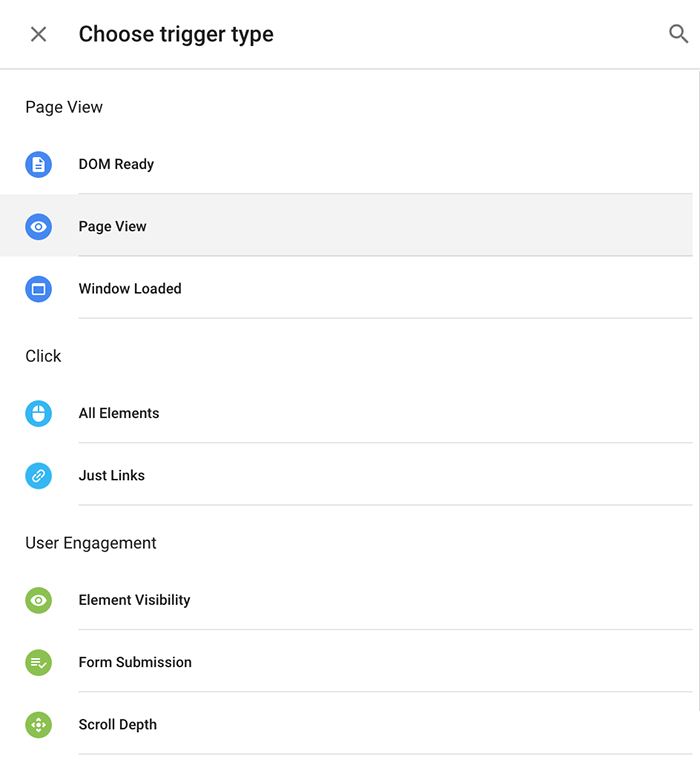This image showcases a settings page from an unidentified software program. The page is designed for configuring triggers and features minimalistic aesthetics with a sparse layout, offering options without detailed descriptions. 

At the top, there is a search bar with the text "choose trigger type" entered. To the left of the search bar, an 'X' icon is visible, while a magnifying glass icon for search is located to the right. 

Below the search bar are search results categorized under different headings:
- **Page View**: Includes options such as DOM Ready, Page View (currently highlighted), and Window Loaded.
- **Click**: Offers the options All Elements and Just Links.
- **User Engagement**: Lists Element Visibility, Form Submission, and Scroll Depth.

Each of these options is accompanied by a small icon, though the page overall lacks detailed explanations for what each trigger does. The interface is clean but minimal, focusing on the selection of trigger types without additional informational guidance.